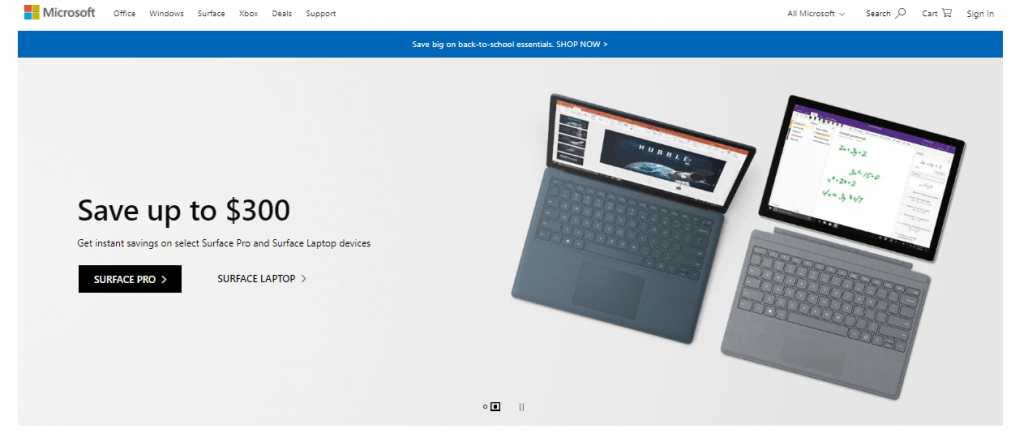**Caption:**

Screenshot from the Microsoft website showing a promotional banner. The top left corner features the Microsoft logo, followed by a navigation menu listing options such as Office, Windows, Surface, Xbox, Deals, and Support. Along the top, there is a blue banner with the text "Save Big on Back to School Essentials" and a "Shop Now" button. Below, there's a large gray box containing an image of two laptops. The laptops are displayed side by side, one in a darker charcoal color and the other in a lighter gray, both showing PowerPoint presentations or graphs on their screens. Accompanying the image, the text states "Save Up to $300 - Get Instant Savings on Select Surface Pro and Surface Laptop Devices." Below this text, there are two clickable buttons: one for the Surface Pro, styled in black, and another for the Surface Laptop, which is unbolded.